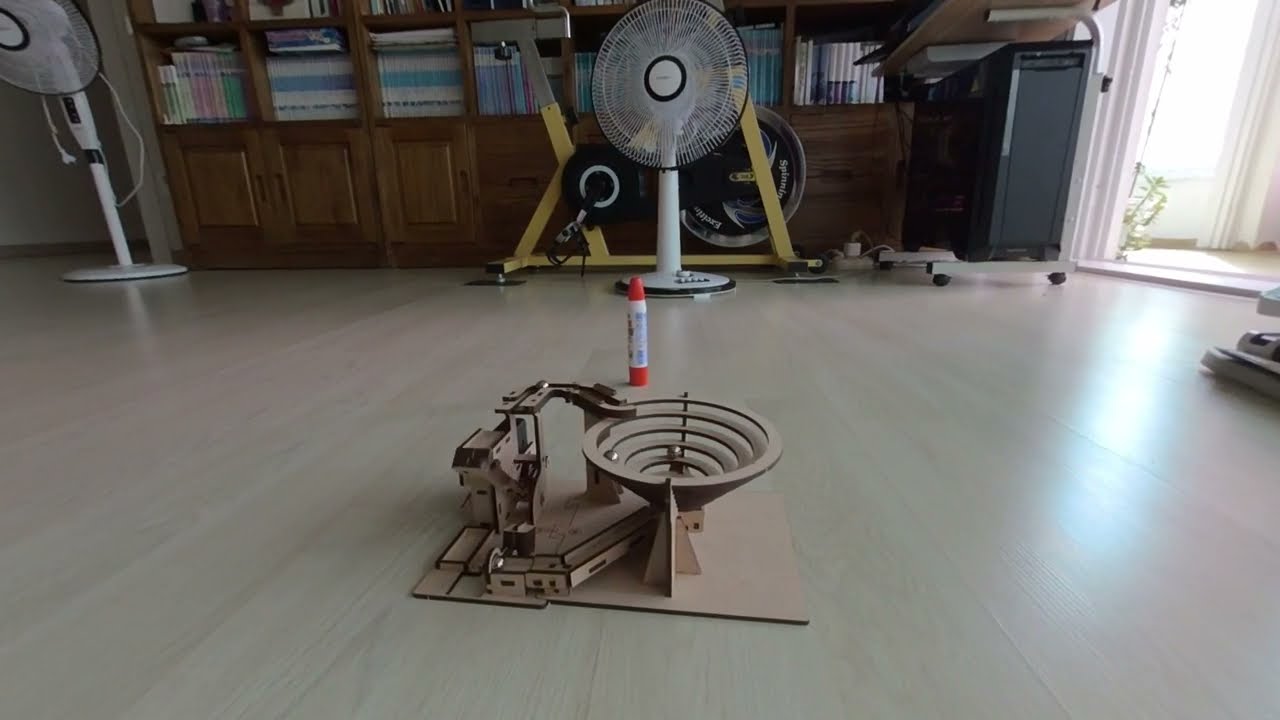The image depicts a sophisticated and intricate robotic machine on a light-colored wood floor comprised of thin strips. The central subject resembles an old-fashioned record player speaker mounted on its side, facing upwards, and a mechanical arm extending over it, connected to a metallic base housing electrical components. This setup forms an inverted triangle or bowl-like configuration, with the structure evoking a complex Rube Goldberg machine. It features a spiral mechanism connected to a funnel with two steel balls inside, suggesting a continuous motion system where the balls spiral down and are then transported back to the top. The context of the scene places this machine in a room that features several background elements: a movable computer desk with a desktop computer, a brown cabinet stacked with manuals, two tower fans (positioned at the corners), and an exercise machine. The setting is well-lit, with sunlight streaming in through a window on the right. The overall ambiance blends a laboratory-like environment with elements of a personal workspace, highlighted by the arrangement of varied apparatus and furnishings.